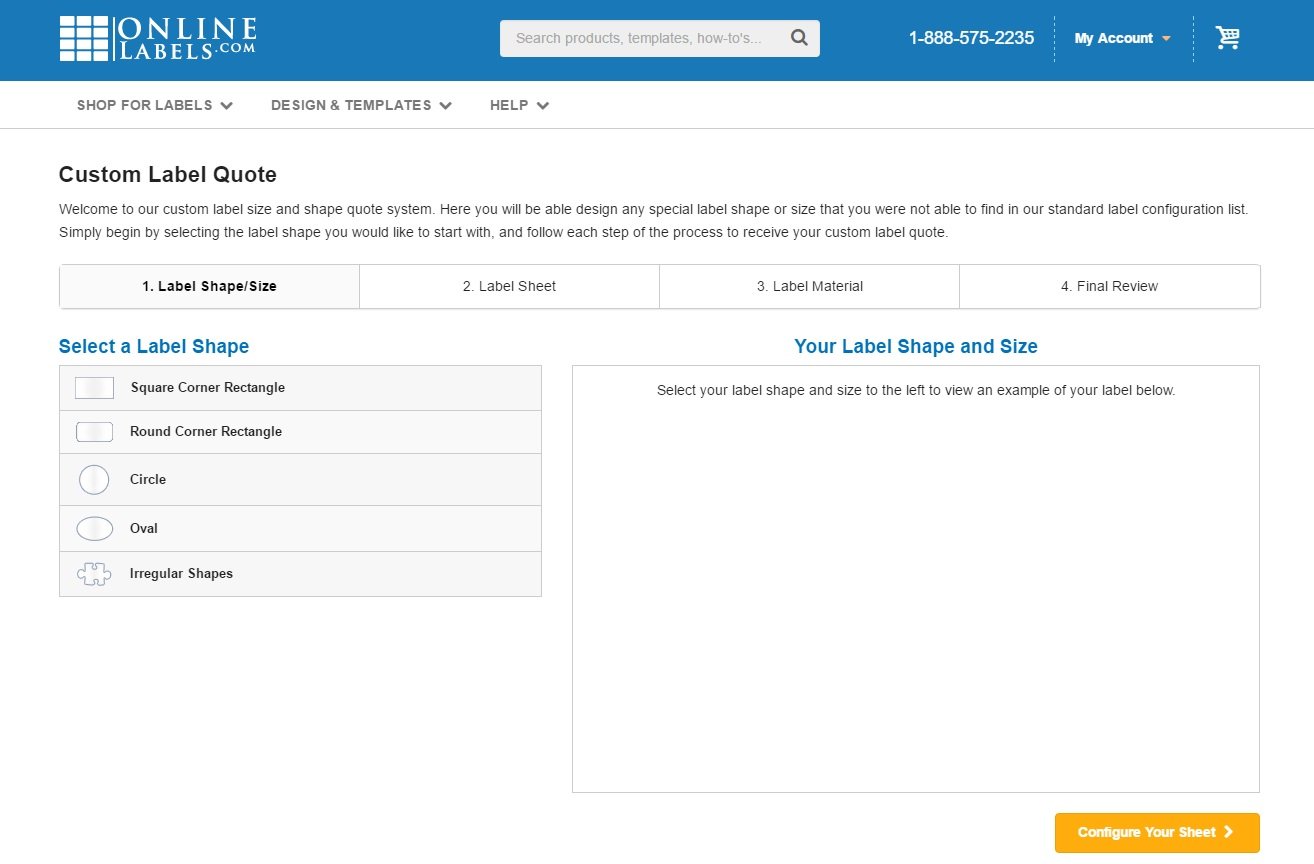The image displays a segment of a website for OnlineFables.com, a custom label quotation service. The website header is designed with a blue strip featuring various options: a search bar for products, templates, and how-to guides. Additionally, there is a phone number, a "My Account" dropdown menu, and a shopping cart icon. Below the header, there are further navigational options including "Shop for Labels," "Design and Templates," and a "Help" button, each with its own dropdown menu.

Prominently displayed in a large font is the title "Custom Label Quote," followed by a welcoming message to the label size and shape quotation system, which allows users to design and customize label shapes. The process is divided into four distinct steps: Label Shape and Size, Label Sheet, Label Material, and Final Review. The image illustrates step one: Label Shape and Size. 

In this step, users can select various label shapes, such as a square-corner rectangle, round-cornered labels, circles, ovals, and irregular shapes. To the right, there is a section to select and view an example of the chosen label shape and size. An orange button labeled "Configure Your Sheet" is positioned beneath these options, indicating the next step in the customization process.